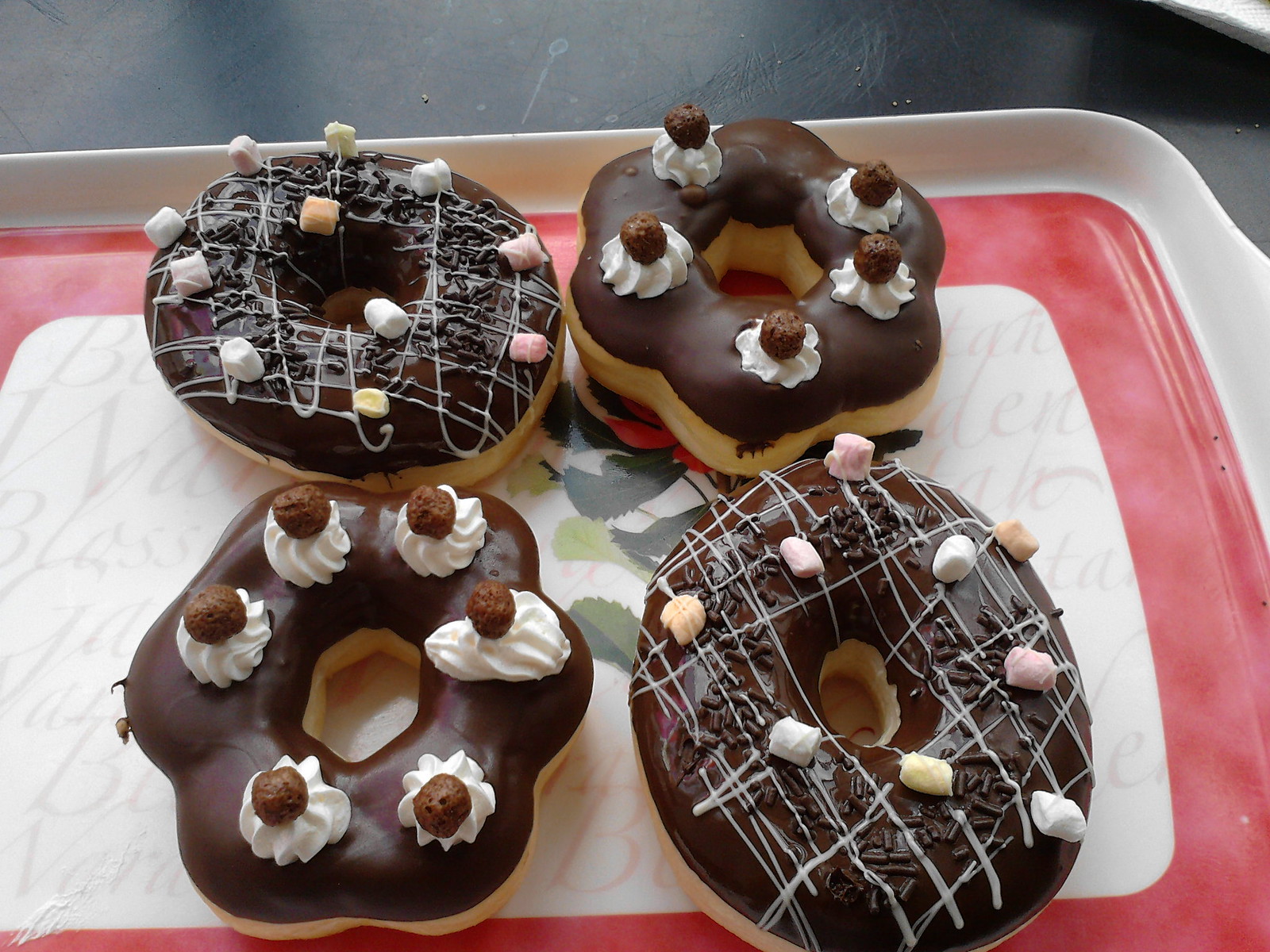A white rectangular tray with a thick red trim and an inner section featuring unreadable text and green leaf designs holds four uniquely adorned doughnuts. Two of the doughnuts are round with chocolate frosting, crisscrossed with white icing, and topped with colorful mini marshmallows (pink, yellow, green, and tan) and chocolate sprinkles. The other two doughnuts have a distinctive flower shape with chocolate frosting, each decorated with small dollops of whipped cream and topped with chocolate balls akin to Cocoa Puffs. The arrangement is set against the backdrop of a black table with visible scratches, suggesting a quaint, perhaps artisanal cafe atmosphere.